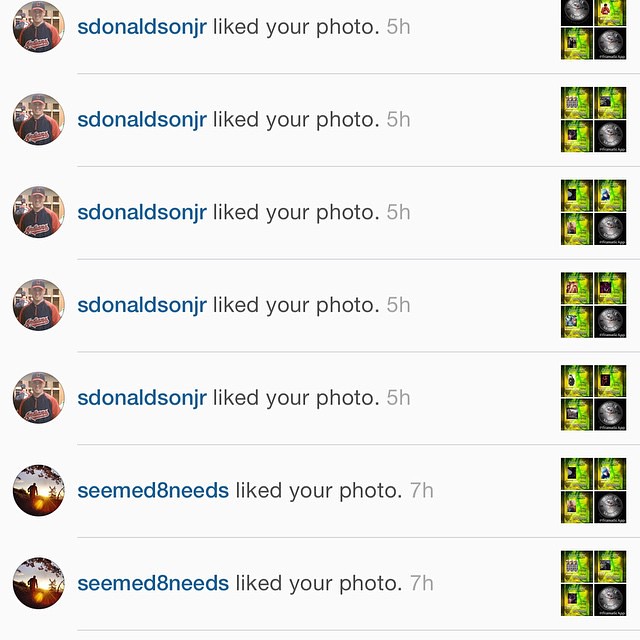This color screenshot, likely from a social media site like Instagram or Facebook, shows a vertical, predominantly square-formatted list of users who liked various photographs. The page is designed to display who liked the photos and when, with no specific site branding visible. Notably, S. Donaldson Jr. liked multiple photographs within the last five hours, while another user, "Seemed8needs," liked several photographs about seven hours ago. Each user’s profile picture is displayed inside a circular frame to the left of their name, which is written in blue text. To the right of each name, in black text, is the duration since they liked the photos, with miniature compilations of four small, color-varied photographs accompanying these details. The images within the screenshots are perhaps linked to an adult-oriented club in Cleveland, Ohio. The overall format and style are typical of social media updates viewed on a smartphone, as the layout is vertically oriented.